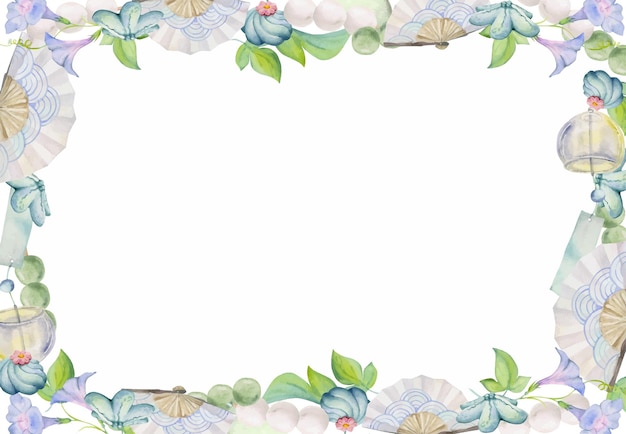The image depicts a rectangular decorative border, ideally suited for use as a template for stationary or an invitation card. Set against a landscape orientation, the border features an intricate design that combines various natural elements. Predominantly light tans, blues, purples, and greens create a subtle, faded color palette that evokes a serene, almost vintage feel.

The border showcases a diverse array of elements: green leaves, light-colored seashells, and white and blue fans. Additionally, there are pearls, some white and some green, enhancing the ornate appearance. Among the features are also purple-bloomed flowers, vines, and glass-like spheres that appear mirrored and positioned twice within the frame. Some details like a starfish-like green flower and a design resembling the icing of a cupcake with a little flower on top add to the overall charm.

The perimeter elements—such as semicircular patterns in blue, white, and dark accents—contribute to the frame's fanned-out and elaborate design, making it an ideal, aesthetically pleasing choice for a garden party invitation or any other elegant, decorative use.